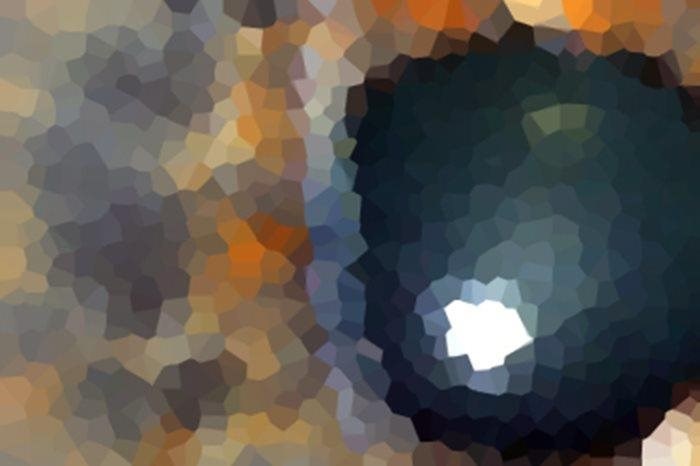This image depicts an abstract and colorful mosaic-like painting or digital artwork, characterized by its out-of-focus clusters and rock-like formations. These clusters, composed of a variety of hues including greys, greens, yellows, oranges, tans, and multiple shades of blue, span from the left to right of the picture. Towards the right side, a prominent feature emerges - a circular, eye-like shape with a black and bluish outer ring, transitioning to grey in the center, and culminating in a solid white opening at the bottom. The left side of the image predominantly showcases earthier tones, such as browns and dark oranges, adding to the mosaic’s dynamic color palette. The overall impression is of a vibrant, textured design that blends an array of colors and shapes, suggesting a sense of depth and randomness within the pattern.